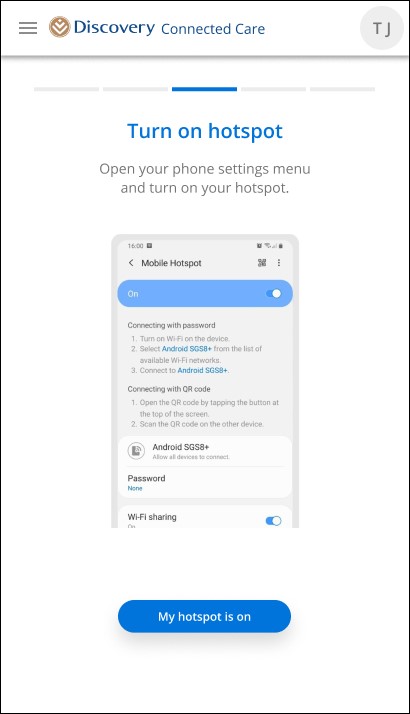The image depicts a webpage from the Discovery app focused on connected care features. At the top, a blue header reads "Discovery Connected Care," accompanied by the Discovery logo in brown and white, a menu icon on the top left, and a profile icon labeled "CJ" on the top right.

Below the header are five horizontal grey lines, with the center line highlighted in blue, displaying the text "Turn on Hotspots." Beneath this, instructional text in grey advises the user to "Open your phone settings menu and turn on your hotspots." 

Accompanying the instructions is an image of a mobile phone with a grey screen indicating "Mobile Hotspots" with a toggle switch turned on against a blue background. The screen reads "Connecting with Password," followed by three steps: 
1. Turn on Wi-Fi on the device,
2. Select "Android SGS 8 Plus" from the list of available Wi-Fi networks,
3. Connect to "Android SGS 8 Plus."

Another section titled "Connecting with QR Code" instructs users to:
1. Open the QR code by tapping the button at the top of the screen,
2. Scan the QR code with another device,
3. Allow all devices to connect with the "Android SGS 8 Plus" (Password: none, Wi-Fi sharing: on).

At the bottom of the page, there is a blue button labeled "My Hotspot is On."